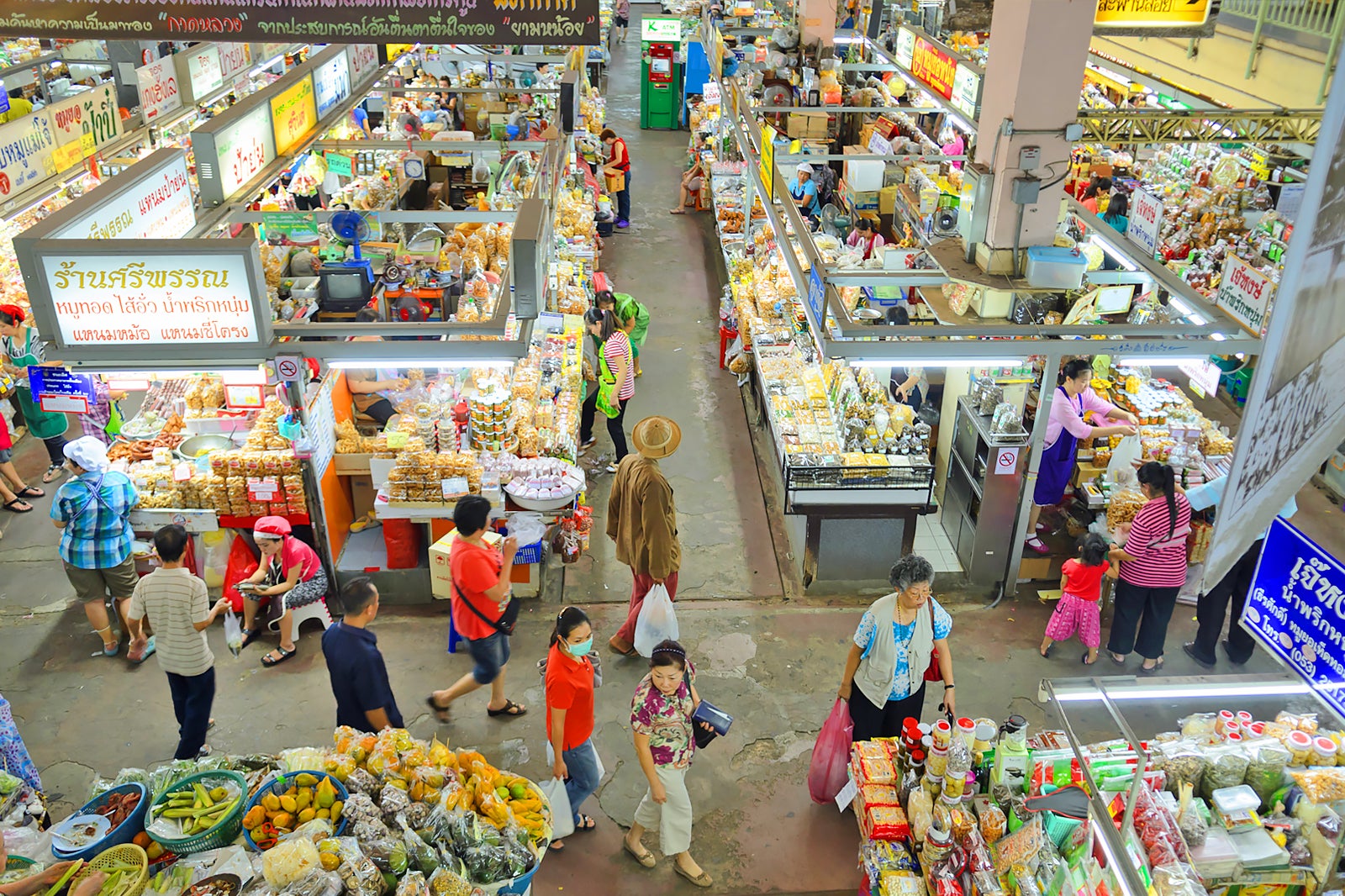This is a vertical, color photograph taken from a high vantage point, providing an expansive overhead view of the bustling interior of a grocery store, possibly located in Thailand. The gray concrete floor is visible beneath numerous rows of shelves and open-refrigerated containers brimming with a variety of products. The shelves, with gray bodies and white tops, display an assortment of foods, including fresh produce, jars, and bread. Various food stalls and packaged foods occupy the lower left and right corners, respectively.

People of all ages and types, some in masks, wander through the aisles, dressed casually in light pants, shorts, and colorful shirts, such as red, blue, purple, and striped patterns. There are men, women, and children, casually dressed, browsing and engaging in their shopping activities. An employee, dressed in a pink top and pink hat, sits on a white stool to the left. Suspended above the scene is a gray metal frame housing lights that illuminate the market.

Signs featuring text in Thai, with colorful palettes of gold, red, white, and blue, add to the vibrant ambiance of the market. The varied colors of the products—from yellow and green to white and purple—contrast with the shoppers’ diverse attire. The expressions on the shoppers' faces reflect eagerness and anticipation, capturing the lively and dynamic atmosphere of this bustling grocery store.